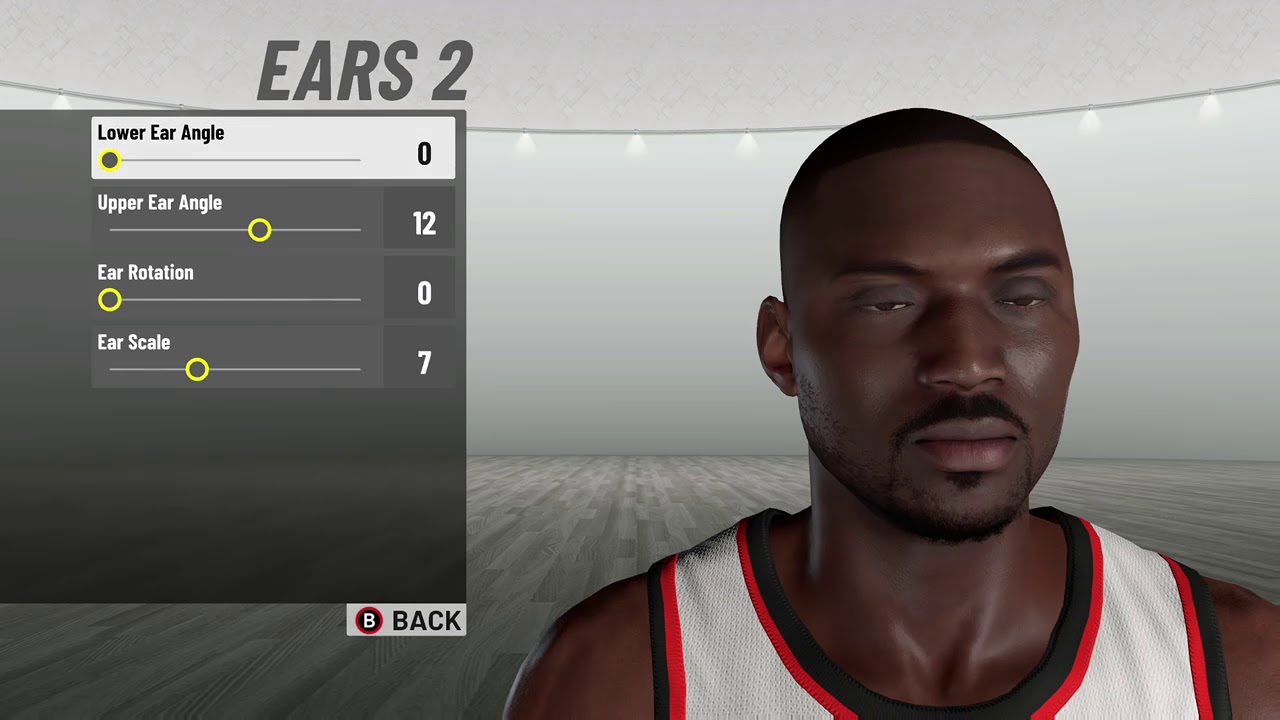A detailed caption for the image could be:

"Screenshot from the 2K basketball video game series featuring the 'Create a Character' screen. The character, a 3D-rendered male with African features, sports short hair and a small mustache and beard. He is wearing a predominantly white basketball jersey accented with black and red. The character occupies the right side of the screen, approximately 60-70% of the space. On the left side, a customization slider titled 'Ears 2' is visible, with adjustable settings for 'Lower Ear Angle' at 0, 'Upper Ear Angle' at 12, 'Ear Rotation' at 0, and 'Ear Scale' at 7. The background includes well-lit surroundings with wooden flooring, adding to the immersive gaming environment. A 'B' button prompt indicates an option to go back to the previous menu."